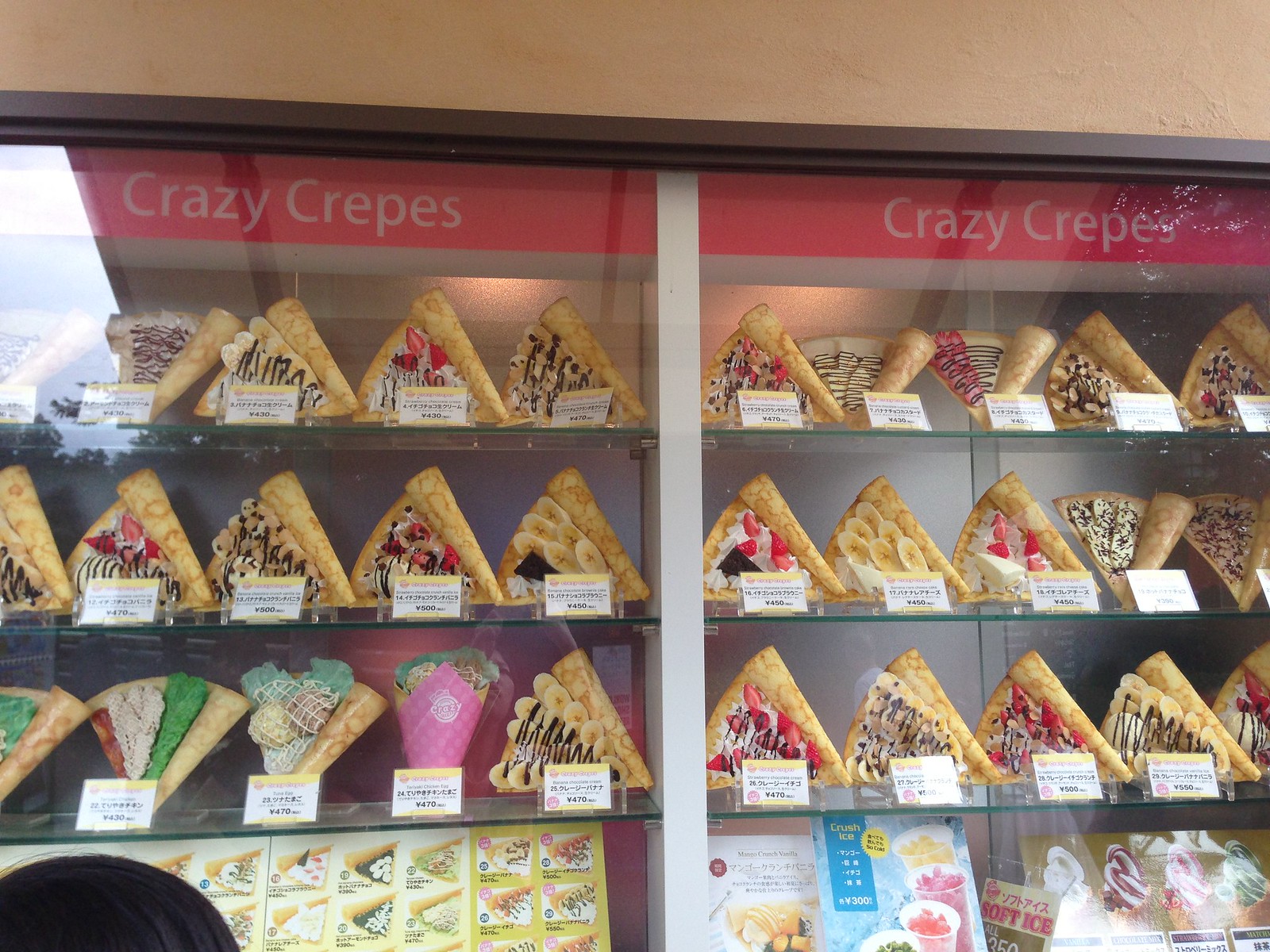This is a color photograph of a glass display case featuring numerous types of crepes in a store. The case is divided into two partitions, each with at least three visible shelves. At the top of both partitions, there's a prominent red bar with white text that reads "Crazy Crepes." The crepes are meticulously arranged in rows of five on each shelf, with around three to four shelves in each partition. Each crepe is partially rolled to form a quarter semi-circle, showcasing an array of colorful fillings at the bottom openings. The fillings vary, including vibrant combinations of strawberries, bananas, chocolate syrup, and white cream, among other toppings. Some crepes also feature unique ingredients like a mysterious green filling and what appears to be cream cheese and bananas. Small placards in front of each crepe display their prices, all written in Japanese. In the bottom right corner of the display, there are ice cream swirls and an ice cream cone, adding yet another tempting option to the array of desserts.